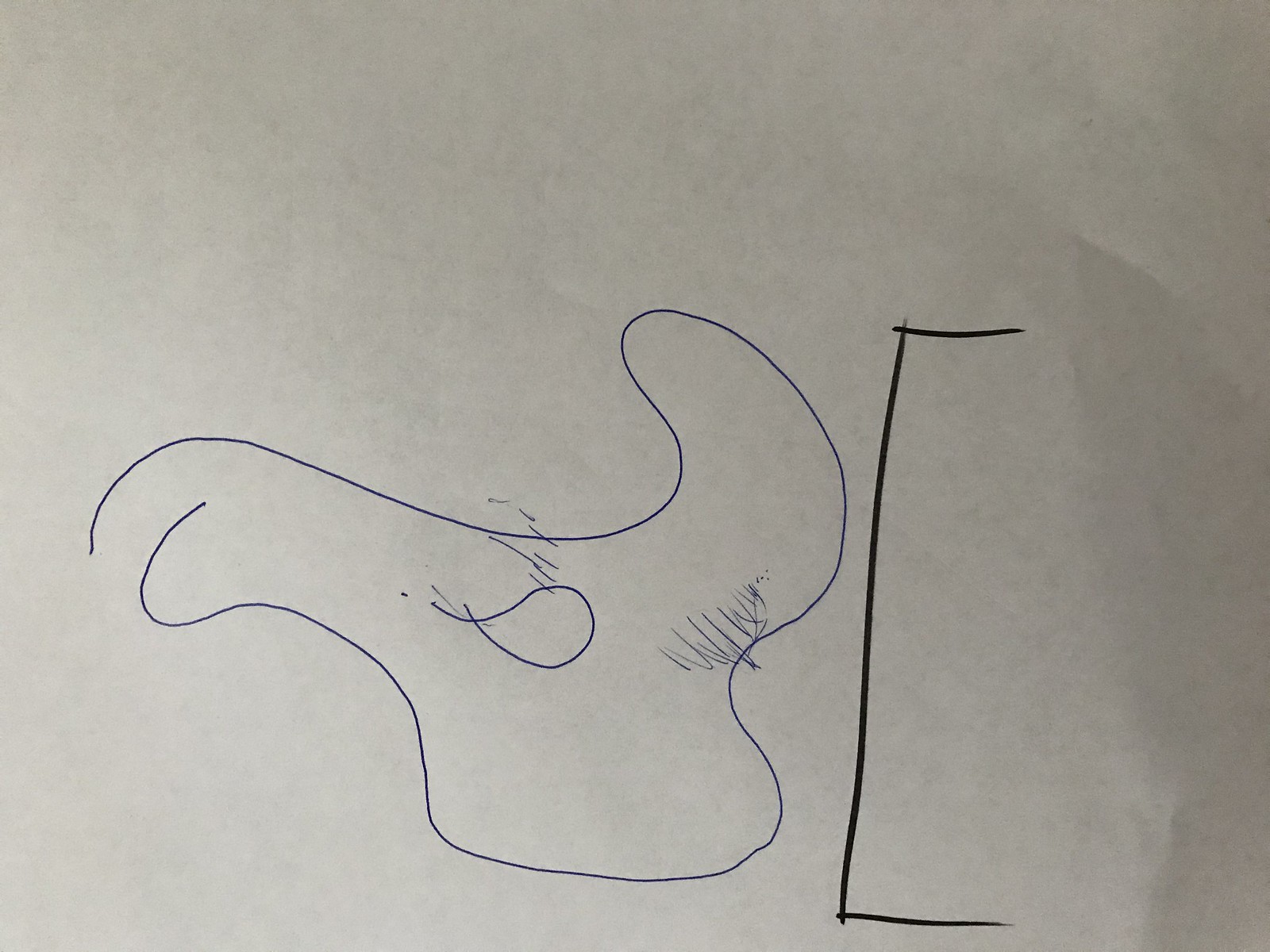The image features a surreal and abstract drawing created using a combination of magic marker and ink pen on parchment-colored paper in a horizontal orientation. Dominating the artwork is an oddly shaped figure positioned from the center to the left. The upper portion of this figure resembles the letter "A," but the legs of the "A" extend downward and curve around to form a shape reminiscent of either a shoe or an elephant with a teardrop-shaped eye. Above and to the right of this eye, several lines add detail, while at the bottom near what would be the heel of the "boot" shape, scribbles provide additional texture.

Adjacent to this whimsical figure is a structure outlined with heavier lines, suggestive of the top of a box-like object. This structure forms a "C" shape with distinct square angles and corners, contributing to the geometric abstraction of the drawing. Despite its intricacies, the overall composition remains enigmatic and does not resemble any particular discernible object, inviting viewers to interpret its forms and patterns freely.